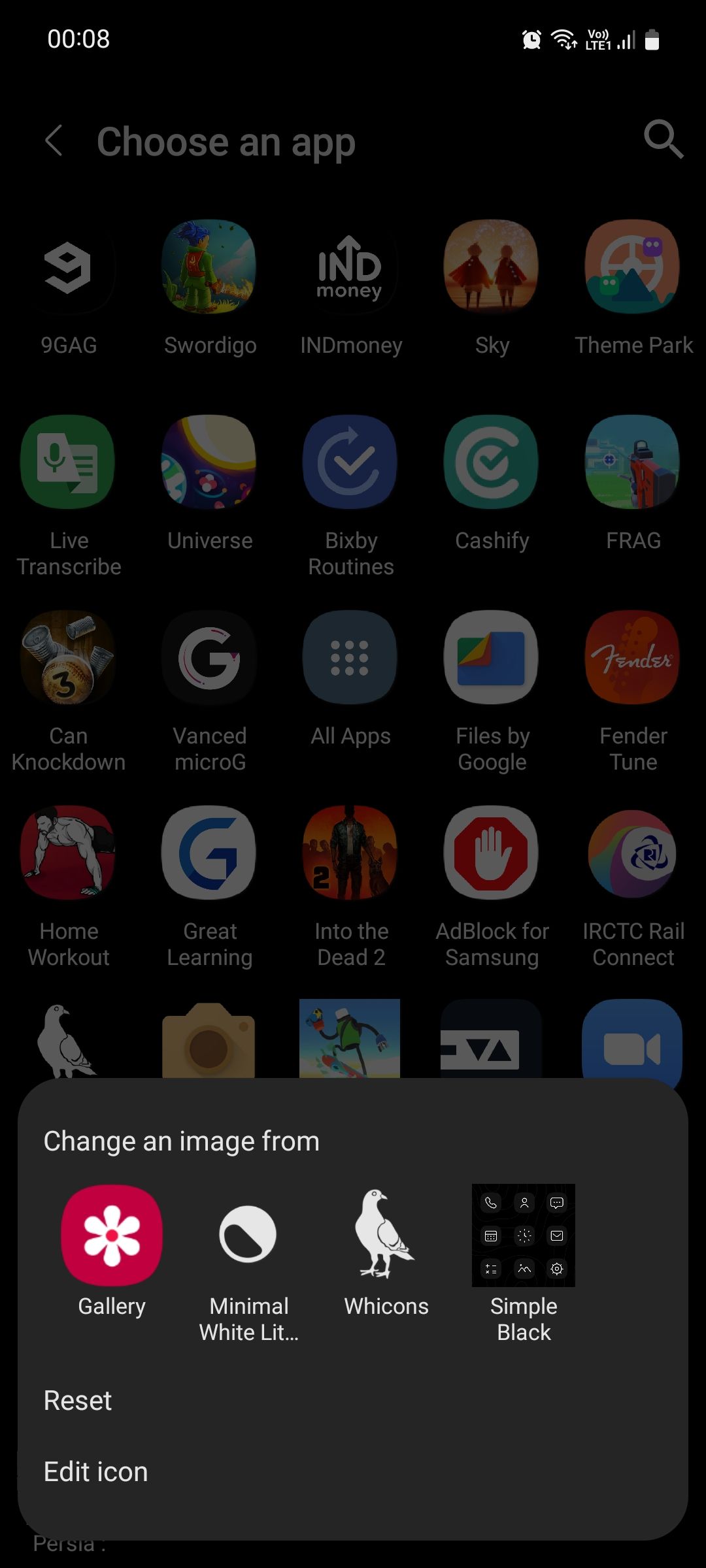This screenshot from a mobile phone, likely running an Android operating system, captures a user interface with a black background. In the top left-hand corner, there is a small white text showing "0.08 times" with standard mobile icons positioned on the right. Below is a partial view of an app list arranged in several rows, with each row containing five app icons. However, the app grid appears greyed out due to an overlaying pop-up box.

The black-background pop-up box, located at the bottom of the screen, is labeled "Choose an app" and includes a search button and a back arrow for navigation. Visible apps in the app grid include: 9GAG, Swordigo, Indmoney, Sky, Theme Park, Live Transcribe, Universe, Bixby Routines, Cashify, Frag, Can Knockdown, Advanced Micro, All Apps, Files by Google, Fender Tune, Home Workout, Great Learning, Into the Dead 2, Adblock for Samsung, and IRCTC Rail Connect. Some app icons are partially obscured by the pop-up box, making their text unreadable. These icons include a bird, camera, cartoon character, triangles, and a blue record button.

The pop-up box displays the text "Change an image from gallery" and features several selectable options, such as:
- A red icon with a flower
- A minimalist icon labeled "LIT"
- A circle divided into half white and half black
- An icon labeled "White climbs"
- An image of a bird
- An option labeled "Simple black"
- A 3x3 matrix of white icons on black

Below these options are a white "Reset" button and a white "Edit icon" option located in the lower left-hand corner of the pop-up box.